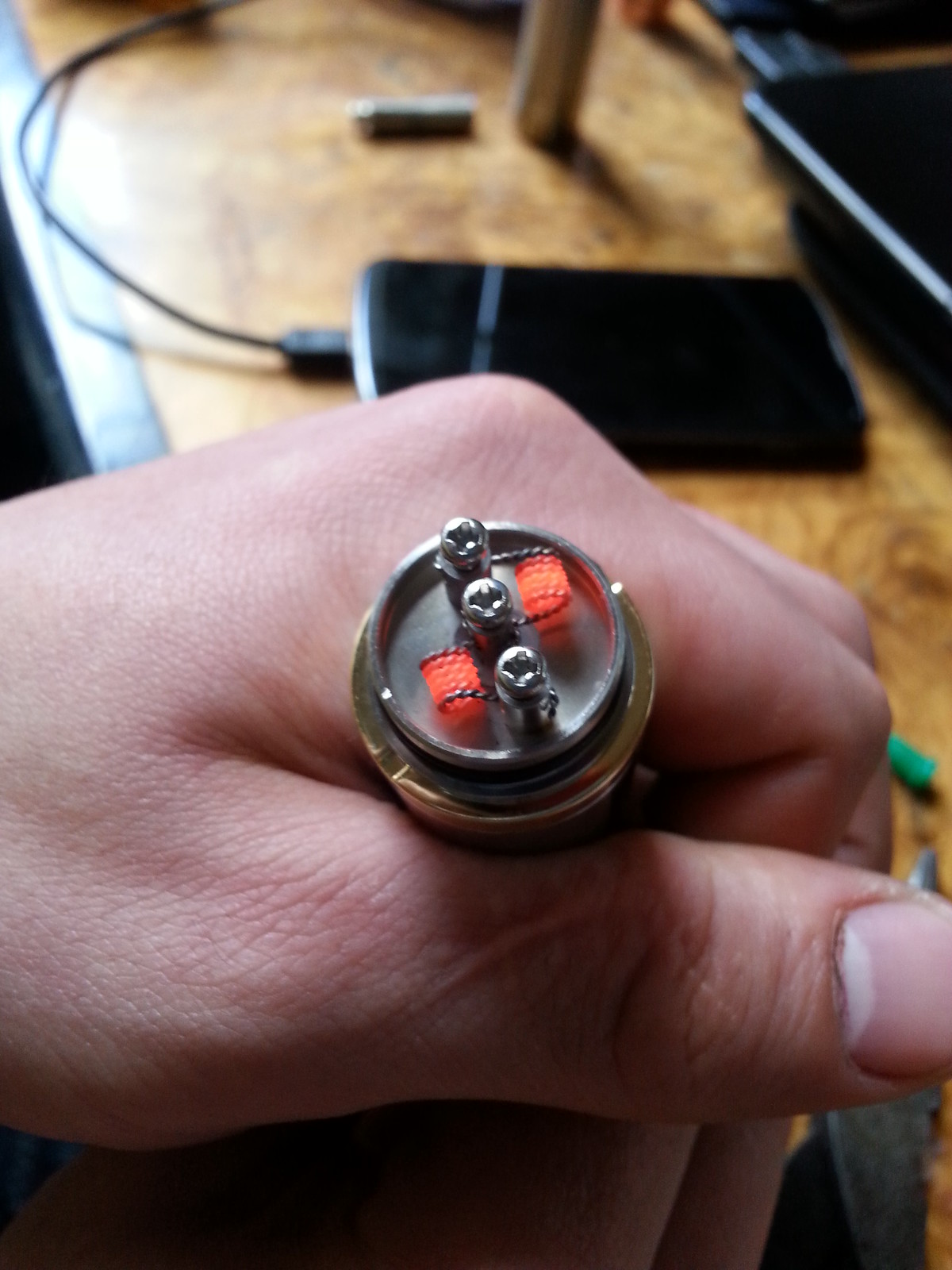In the photograph, a Caucasian person's left hand is prominently displayed in the foreground, holding a small, intricate electronic component. This component is silver and round with a wider gold piece encircling it. It features three Phillips-style screws in a line and two metal coils on either side of the screws that are glowing red hot. The setting appears to be a wooden table or platform. Nearby, a battery and a cell phone plugged into a charger can be seen. Additionally, a black electronic device, which could be a monitor or tablet, is positioned in the top right corner of the image.